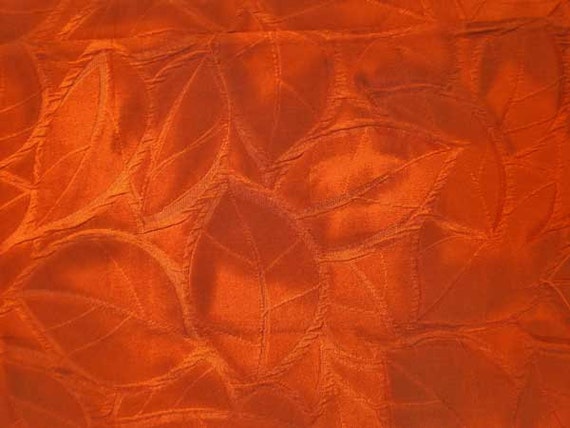This image features a detailed close-up of a piece of fabric adorned with a leaf pattern. The fabric, which occupies the entirety of the frame in a landscape orientation, is primarily colored in shades of orange, with gradients that transition into lighter oranges, yellows, and even hints of red. The leaf pattern appears to be embossed or stamped into the fabric rather than embroidered, providing a textured feel. The leaves, which are scattered throughout the fabric, vary in orientation; those at the top are more densely packed and appear more vertical, while those toward the bottom are more horizontal and spaced out. This intricate design, devoid of any text or signatures, exudes a fall theme, with vivid autumnal colors and natural motifs. The fabric might be part of a decorative item, such as a tablecloth, but its exact purpose is left to interpretation.